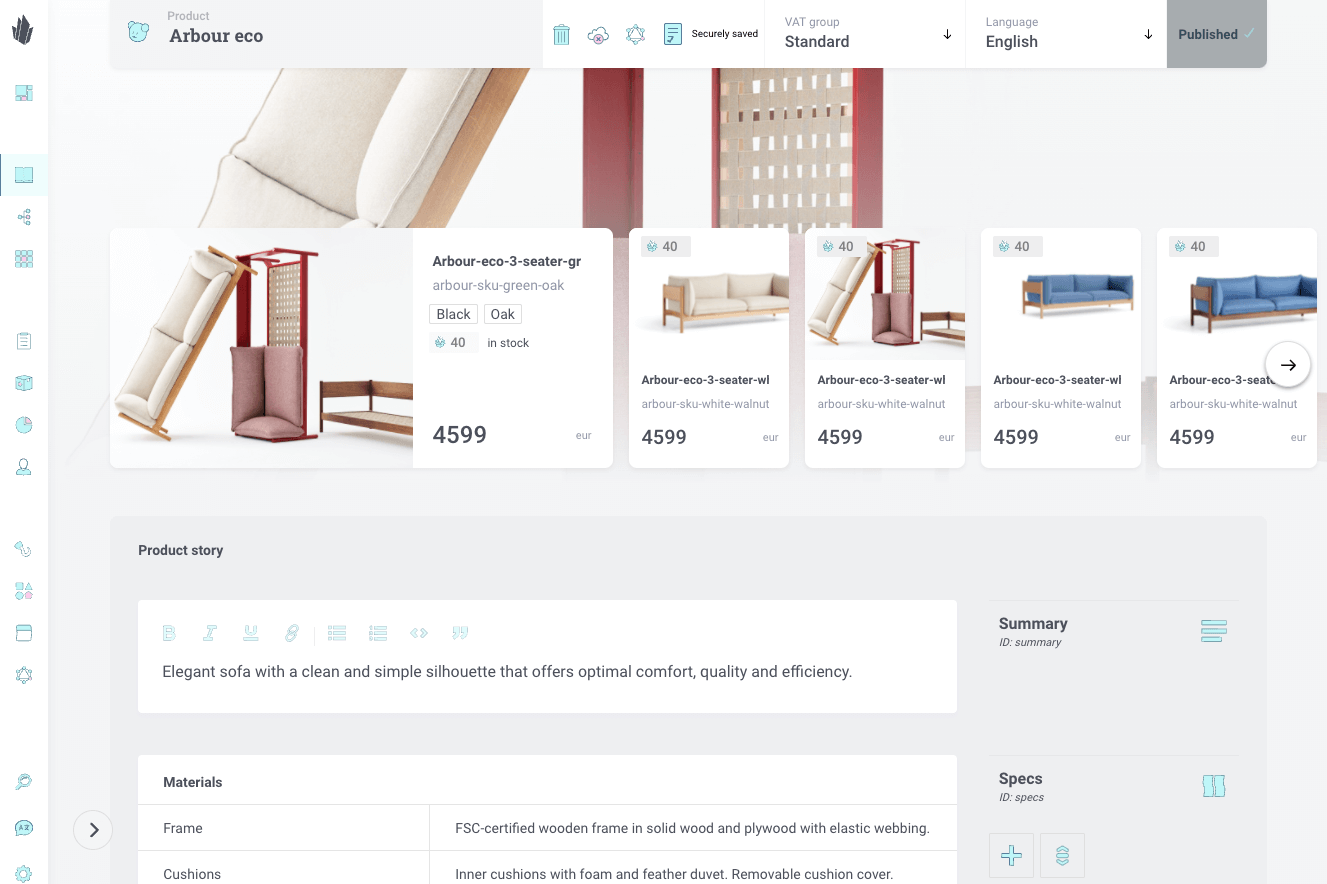This image, sourced from a webpage titled "Arbor ECO," features a user interface displaying various product details. Central to the image is a section where "Arbor ECO" is prominently spelled out, with "Arbor" stylized as "A-R-B-O-U-R". A teal, cartoonish teddy bear head is also visible, adding a whimsical element to the design. Below this, the page lists icons that include a trash can, cloud, star, paper, and a message that reads "securely saved." 

Adjacent to these elements are drop-down menus labeled "VAT group" and "standard," each marked with an arrow pointing downward. Further down, there is a section indicating publication status with the word "published" in gray, accompanied by a teal checkmark.

At the top middle of the page, there are images of couches displayed vertically to reveal their internal structure. This section is labeled "Arbor Echo 3 Seater - GR" and offers options to choose between black or oak finishes, each priced at €4,599. The couches are showcased in various colors including blue, burgundy, and a white-tan mix, providing a visual representation of the available options.